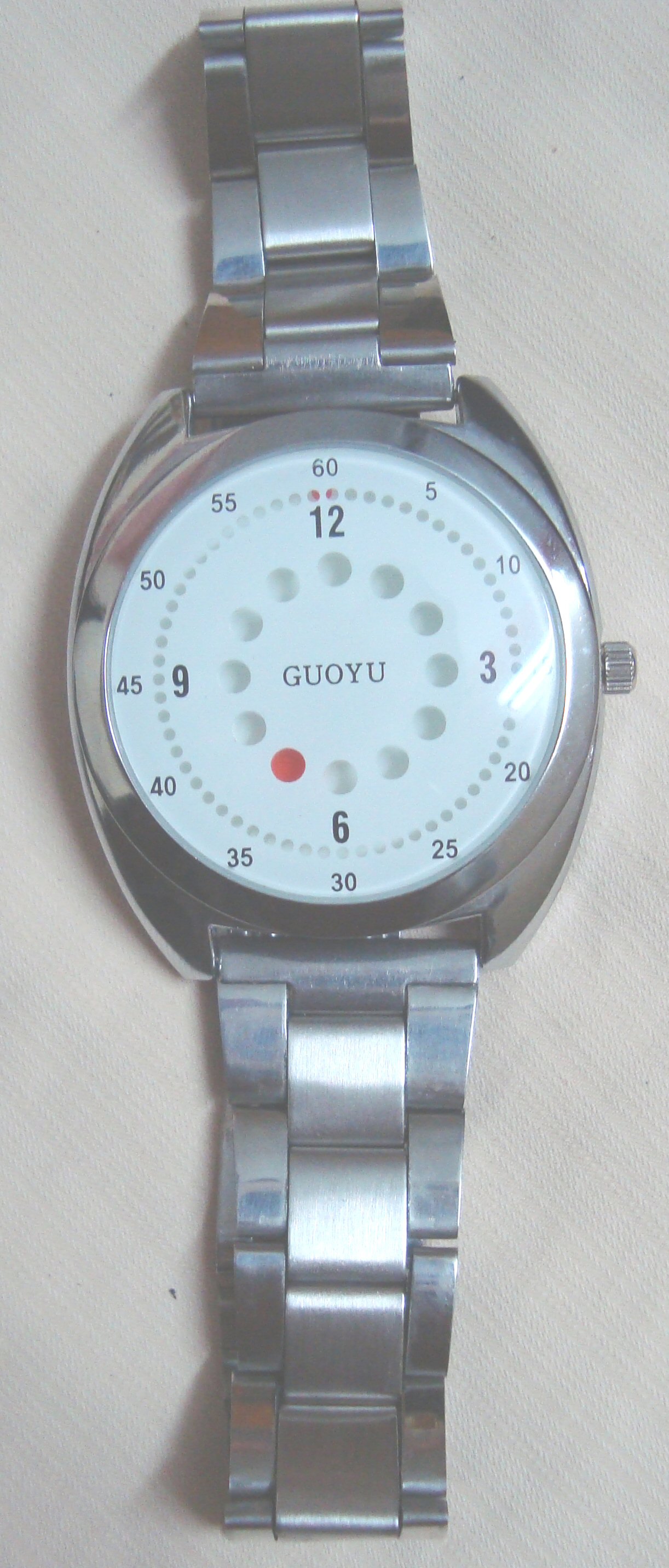The photograph features a wristwatch with a silver or chrome exterior lying on a textured blonde off-white tabletop. The watch has a distinctive design with a white round face. Surrounding the face, the minutes are marked in increments of 5, starting from 60 at the 12 o'clock position down to 5 at the 1 o'clock position, and so forth. The outer ring of the face is perforated with small holes marking each second. Within this outer ring, there are more prominent, larger perforations indicating the 12, 3, 6, and 9 hours, with a notable red dot appearing through the hole at the 7 o'clock position. In the center of the white face, the brand name "GUOYU" is printed in black. A single control knob is located on the right-hand side at the 3 o'clock position. The detailed design and the unique red dot at 7 o'clock contribute to its distinctive aesthetic.